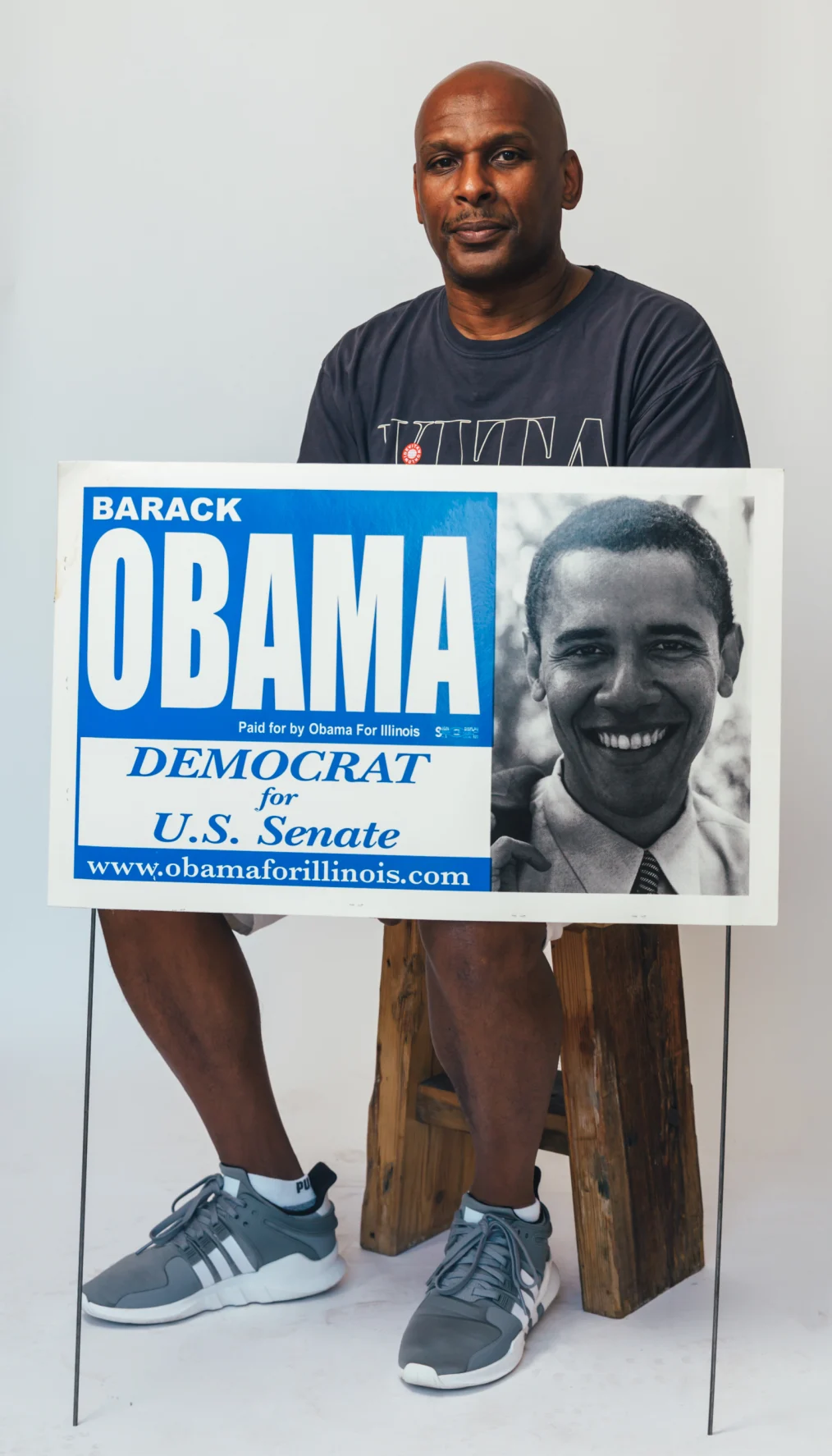In this black-and-white image, a black man with dark brown skin is seated on a wooden stool. He is dressed in a grey shirt with a central logo and grey Adidas sneakers featuring white soles and stripes. The man has short black hair and wears shorts that are partially out of view. He maintains a neutral expression while looking towards the camera. In front of him, held by a stand with two legs, is a prominent blue poster. The poster showcases a youthful black-and-white photograph of Barack Obama, who is smiling and appears to be in his 30s. Obama is depicted wearing a jacket, a white collared shirt, and a tie. The poster text reads: "Barack Obama, Paid for by Obama for Illinois, Democrat for U.S. Senate," with an additional blue rectangle at the bottom bearing the website "www.ObamaForIllinois.com" in white letters. The background of the image is a stark white, highlighting the contrast and central elements of the scene.